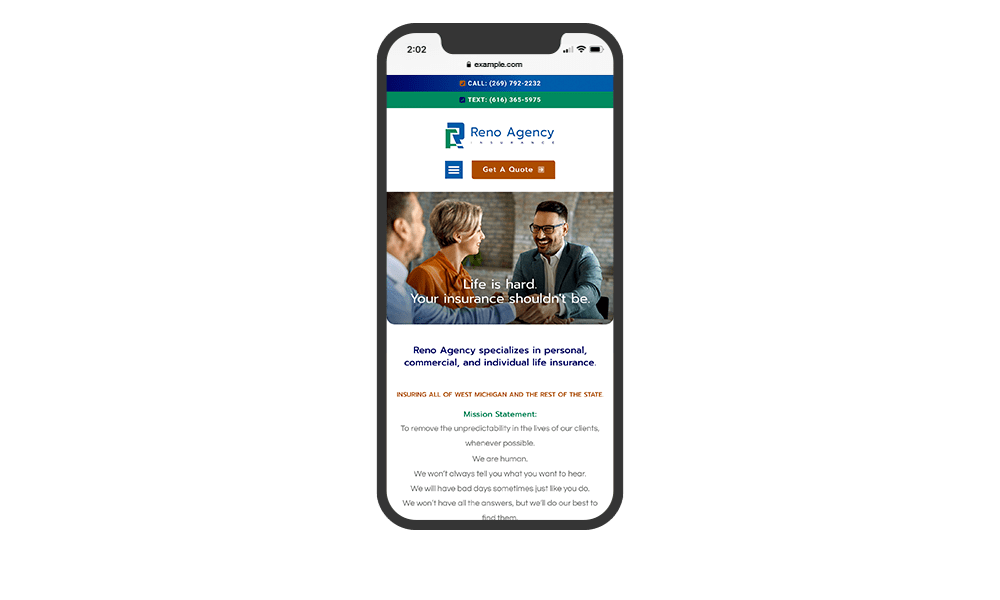This digital representation captures a screenshot of a mobile website, presented in portrait orientation, depicting the interface as seen on a smartphone. The phone's encasement includes a noticeable thicker section at the top for the camera. At the top left, the timestamp shows 2:02 in black text, while the top right shows signal strength (two bars), full Wi-Fi, and a nearly full battery indicator.

Within the topmost white background area, centered black text reads "example.com" accompanied by a small lock icon denoting a secure connection. Below, a blue horizontal bar spans the screen width, featuring white text that reads "Call (269) 792-2232" adjacent to an orange phone icon. Directly below, a green horizontal bar holds white text that reads "Text 616-363-5975" next to a blue phone symbol.

In the main content area, "Reno Agency" is prominently displayed in blue text beside a larger logo consisting of two interlocking 'R's in green and blue. Below, an orange button with white text prompts to "Get a Quote," and to its left, a small blue square with three white horizontal lines indicates a menu button.

The page's visual centerpiece is an image featuring a man in a suit, smiling as he shakes hands with another man on the left, with a woman seated between them, also smiling. Overlaid white text at the bottom of the image states, "Life is hard, your insurance shouldn't be."

Beneath the promotional image, blue text declares, "Reno Agency specializes in personal, commercial, and individual life insurance," followed by another line of orange text, "Ensuring all of West Michigan and the rest of the state." Centered green text labels the section "Mission Statement," followed by gray text down the center conveying the statement: "To remove the unpredictability in the lives of our clients. Wherever possible. We're human. We won't always tell you what you want to hear, we will have bad days sometimes just like you do. We won't have all the answers, but we'll do our best to find them."